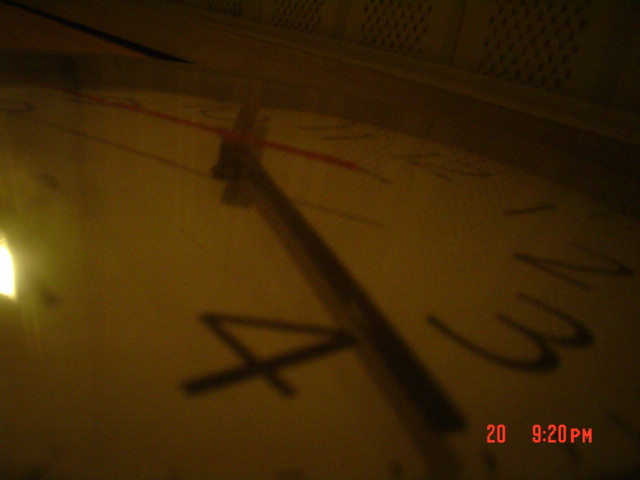In this image, we see a clock taken from an unusual and slightly disorienting angle, with the camera appearing to be upside down and angled from the right side of the clock. The image is quite dark and blurry, with a weird yellow light on the left-hand side. The wooden clock has a glass protective cover over its black numbers. The clock's most visible numbers are 3 and 4, with both the hour and minute hands positioned between these numbers, indicating the time is about 10:18. The red second hand is thin and distinct, positioned around the 8 or 9. The numbers from 4 to 9 are cut off in the image, but from this perspective, the eye moves directly from the 4 across to the 10. Additionally, there is a red digital timestamp at the bottom reading "20, 9:20 p.m." In the background, white locker doors with small holes can be made out, adding to the overall dim and cluttered ambiance of the image.